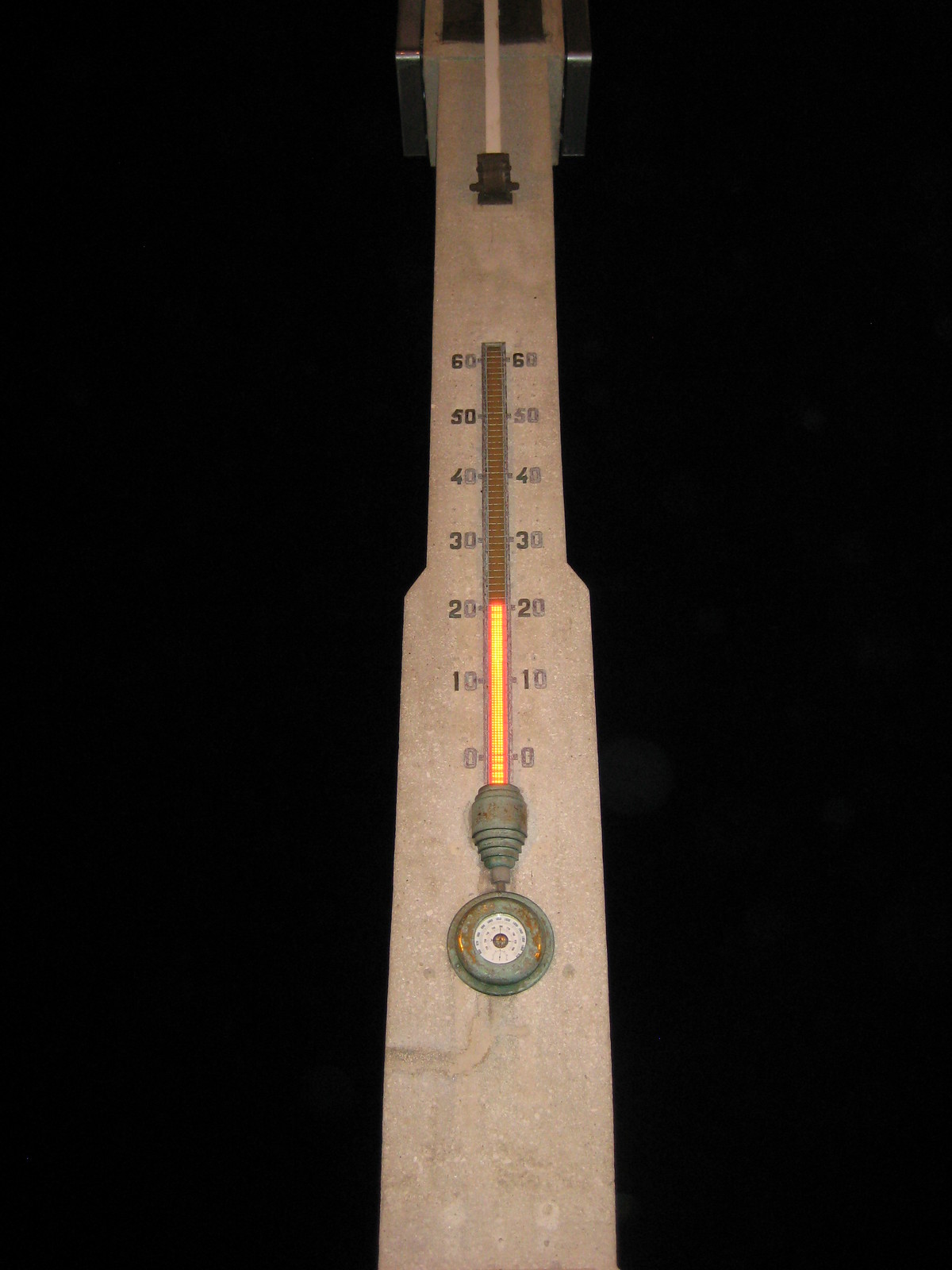The image depicts a thermometer with a range from 0 to 60 degrees Celsius. The temperature scale is marked in increments of 10 degrees, with numbers in both red and black text displayed on the left and right sides, respectively. The thermometer's mercury column is red and currently indicates a temperature of approximately 21 degrees Celsius. The bottom of the thermometer features a circular design with a small green element near the 0-degree mark. At the top, there is a distinct marker, with black detailing running along both the left and right edges of the thermometer.